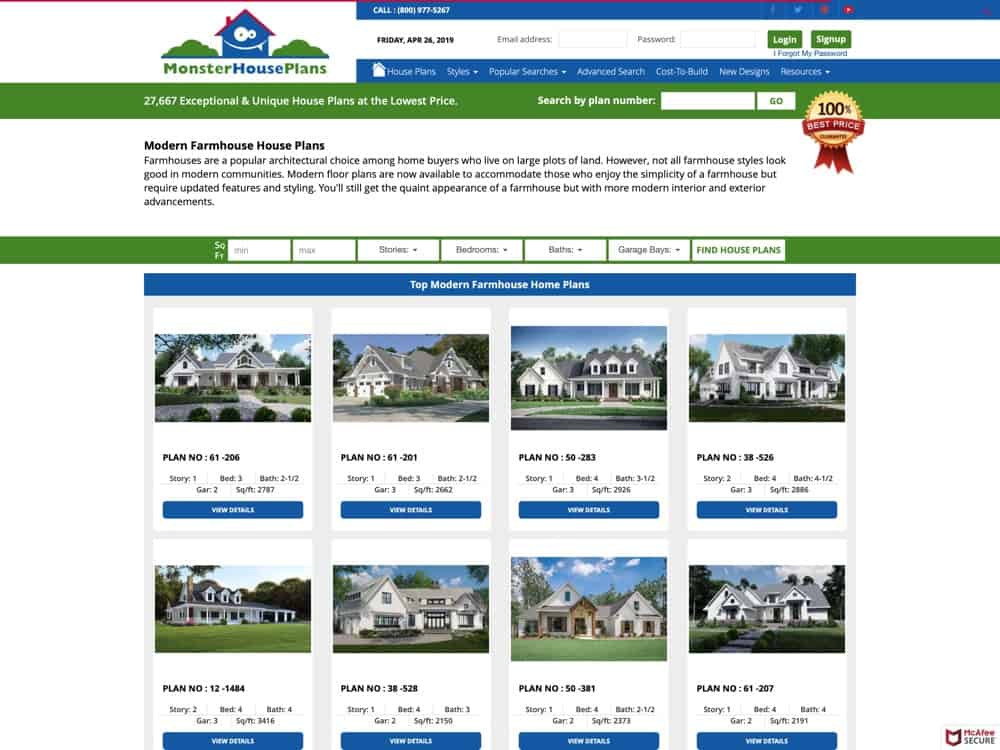The website "Monster House Plans" features a quirky logo depicting a whimsical house with a face, surrounded by two bushes. Scrolling down the page reveals a section dedicated to Modern Farmhouse House Plans. These plans cater to homeowners who favor the rustic charm of a farmhouse but with contemporary design elements, making them suitable for both rural and modern suburban settings.

The site describes how traditional farmhouses are popular among those with large plots of land but notes that not all farmhouse styles fit well in modern communities. The modern farmhouse plans bridge this gap by blending classic farmhouse aesthetics with updated floor plans and conveniences.

Displayed are various house designs, each boasting expansive lawns, gray roofs, and white walls, giving the community a cohesive suburban feel. The houses vary in the number of bedrooms and bathrooms but share a similar architectural style, making them appear somewhat interchangeable. The homepage includes a search bar at the top, along with options for users to log in and customize their browsing experience.